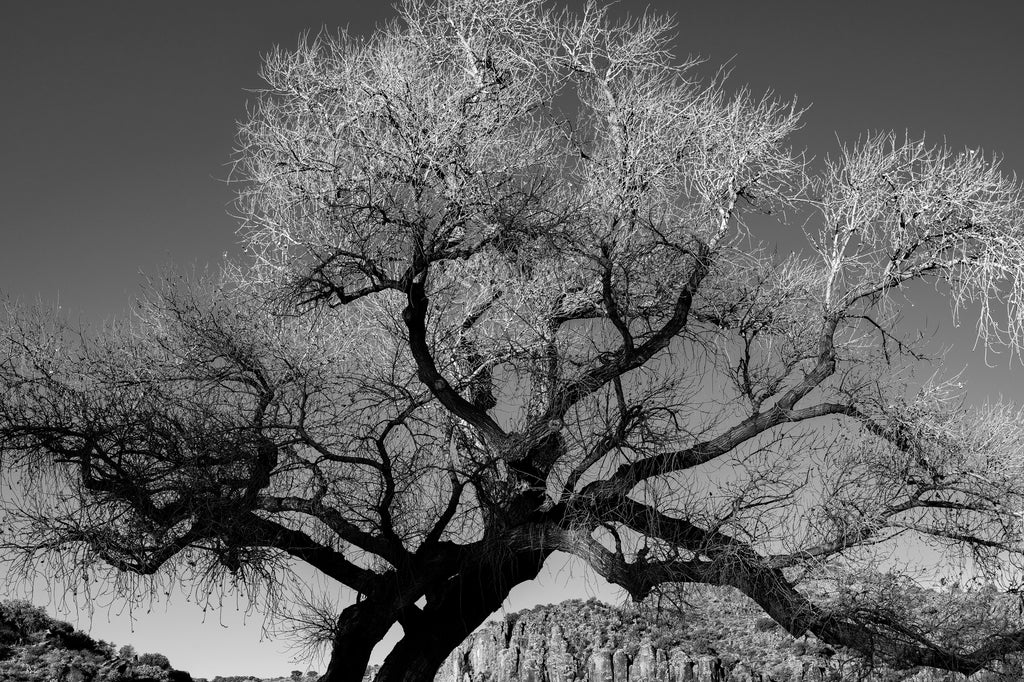This captivating black-and-white image, evocative of an Ansel Adams photograph, showcases an exceptionally large and ancient tree with a thick, sprawling trunk that appears almost sculpted by time. The trunk, prominent and darker at the base, gradually lightens towards the top, giving the impression of an ombre effect that mirrors the transitioning tones of the sky. The tree's myriad of branches extend in all directions, devoid of leaves, suggesting a winter or late fall scene. At the top, the branches appear almost white, resembling snow-covered limbs, although it's likely due to the lighting in the photograph rather than actual snow. The sky behind the tree transitions from a light gray at the horizon to a darker gray higher up, adding to the dramatic effect of the image. Beneath the tree, the landscape features a rocky terrain that hints at a desert environment, possibly resembling the flat-topped rock formations of Arizona or New Mexico. The overall composition, with no people or text, focuses entirely on the tree and its stark beauty against the varied shades of the sky, capturing a timeless and serene moment in nature.